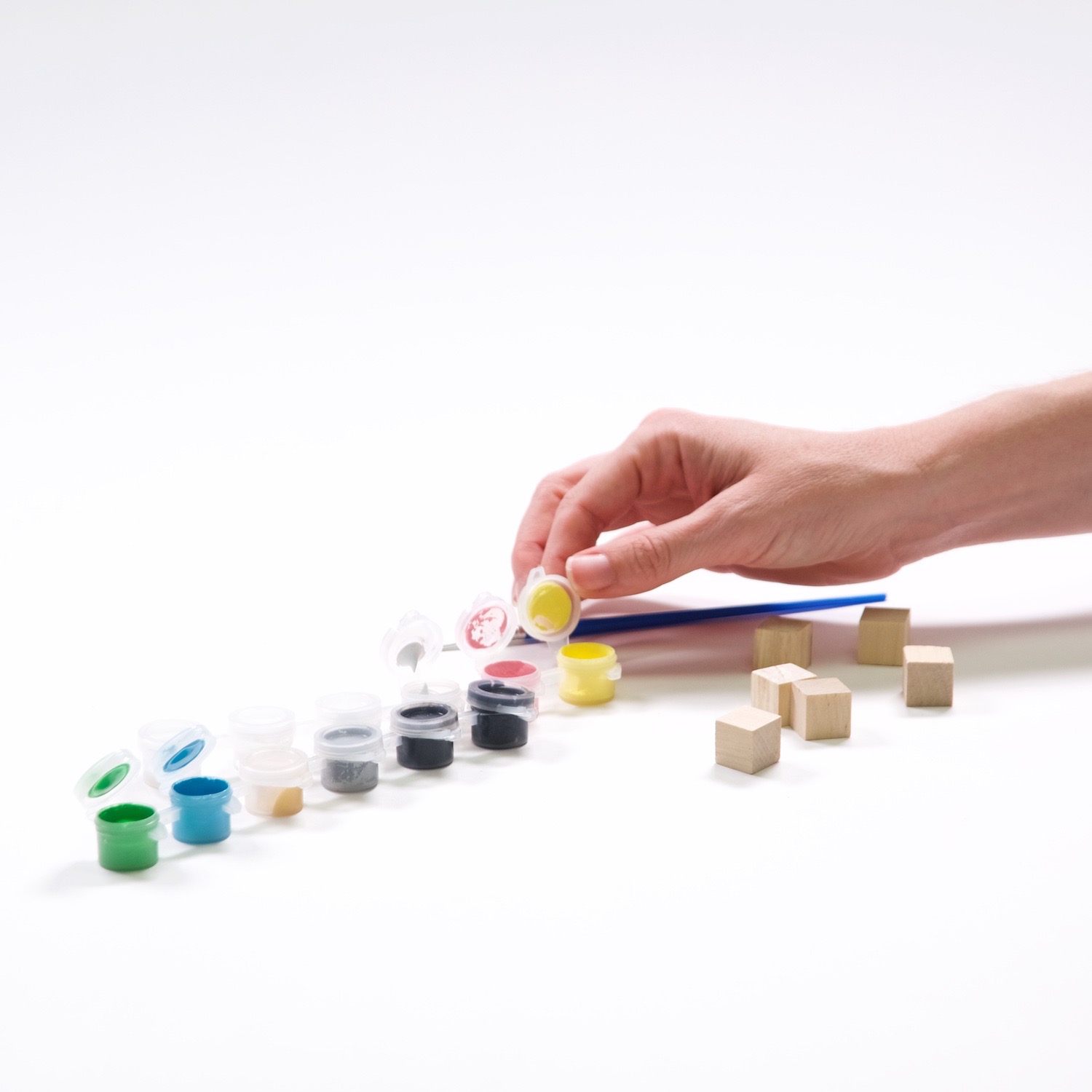This color photograph in a square format captures a DIY art setup. At the center right of the image, a right-handed white person is holding the lid of an open pink acrylic paint pot between their thumb and index finger with their palm facing down. The paint pots, arranged in two rows from right to left, contain assorted colors: pink, two blacks, gray, yellow, blue, and green. Some of these pots are open while others are closed. In addition, there is a blue-handled paintbrush lying horizontally beneath the hand. To the right, under the person's hand, are six unpainted cube-shaped wooden blocks, similar in size to the paint pots. The background features a light gray gradient, darker at the top and almost white at the bottom. The colors in the scene include light gray, white skin tones, light brown, yellow, black, gray, blue, and green, giving it a vivid yet realistic appearance. The image embodies a photographic realism style and focuses purely on the tools and material for a miniature paint project, with no text or numbers distracting from the view.